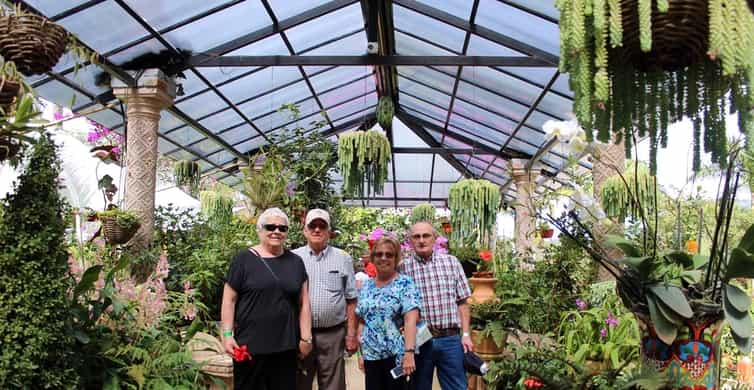In this photograph, four individuals, likely two older couples, are standing in what appears to be a nursery or a greenhouse filled with potted and hanging plants. The structure has a glass or tinted plastic roof with open sides, supported by ornate pillars, allowing light to filter through.

Starting from the left, the first woman has short white hair and wears black pants with a black shirt. She accessorizes with sunglasses and a green bracelet and holds a red flower. Next to her stands a man in a plaid collared shirt, brown shorts, and a ball cap.

To his right, the second woman has short light brown hair and wears a blue floral shirt, black shorts, and glasses, while holding a phone in her hand. Lastly, the fourth individual, an older man with a receding hairline, wears a plaid button-down shirt, blue jeans, a belt, glasses, and holds a hat in his hand.

The image, likely taken for a personal photo album, showcases the casual and relaxed atmosphere of the greenhouse, with its lush greenery providing a vivid backdrop.